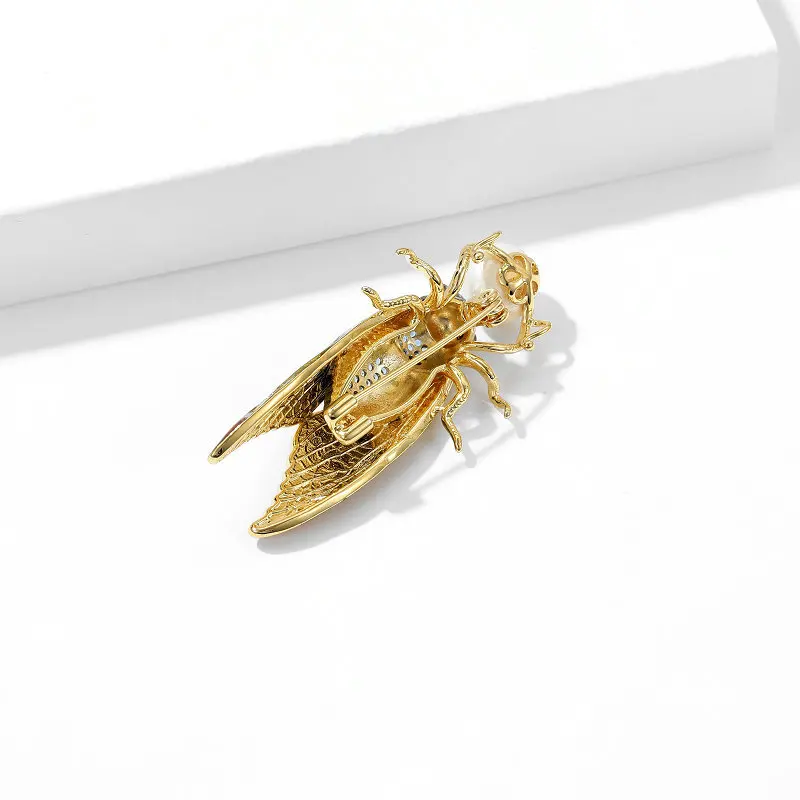The image showcases a detailed gold pin designed in the shape of a winged beetle, set against a white blotchy background that varies slightly in shades. The beetle is positioned upside down, revealing a long, thin gold clasp on its back. This intricate piece of jewelry features six legs, with the front two legs delicately holding a round gold object. Additionally, the beetle’s head is accentuated with a diamond, and there are smaller diamonds adorning its back. The beetle's wings are denoted with a darker, brass-like tone, contrasting with its gold legs, head, and body. A subtle shadow is cast under the pin from a raised white platform on the left, contributing to the overall three-dimensional effect. The pin, approximately two inches long, rests near a white box, adding a grayish hue to parts of the background due to the interplay of light and shadow.